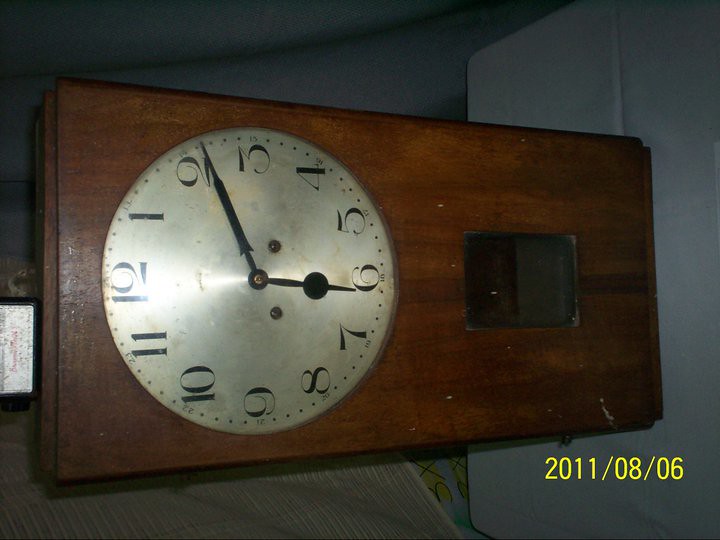In the photograph, an old walnut clock, rectangular in shape, lies on its side. The clock face, positioned in the top half of the wooden frame, showcases a distinct Art Deco style with clear black numbers in a standard format, not Roman numerals, on a silver background. The hour hand points to 6, while the minute hand is between 2 and 3. The slightly tarnished silver face contrasts with the dark wood frame. The clock also features a small slot at the bottom center of the wood frame. 

The scene is captured with a predominantly gray background, possibly a wall, creating a stark contrast with the dark wooden clock. The image is taken from a side angle, presenting the clock in a unique perspective. There is a noticeable shadowed area suggesting a white table with subtle indentation lines below the clock, and some tan fabric is visible behind it. A date stamp at the bottom right of the photo reads "2011-08-06," or alternatively "06-08-2011," denoting the precise date the picture was taken, casting slight ambiguity depending on the date format.